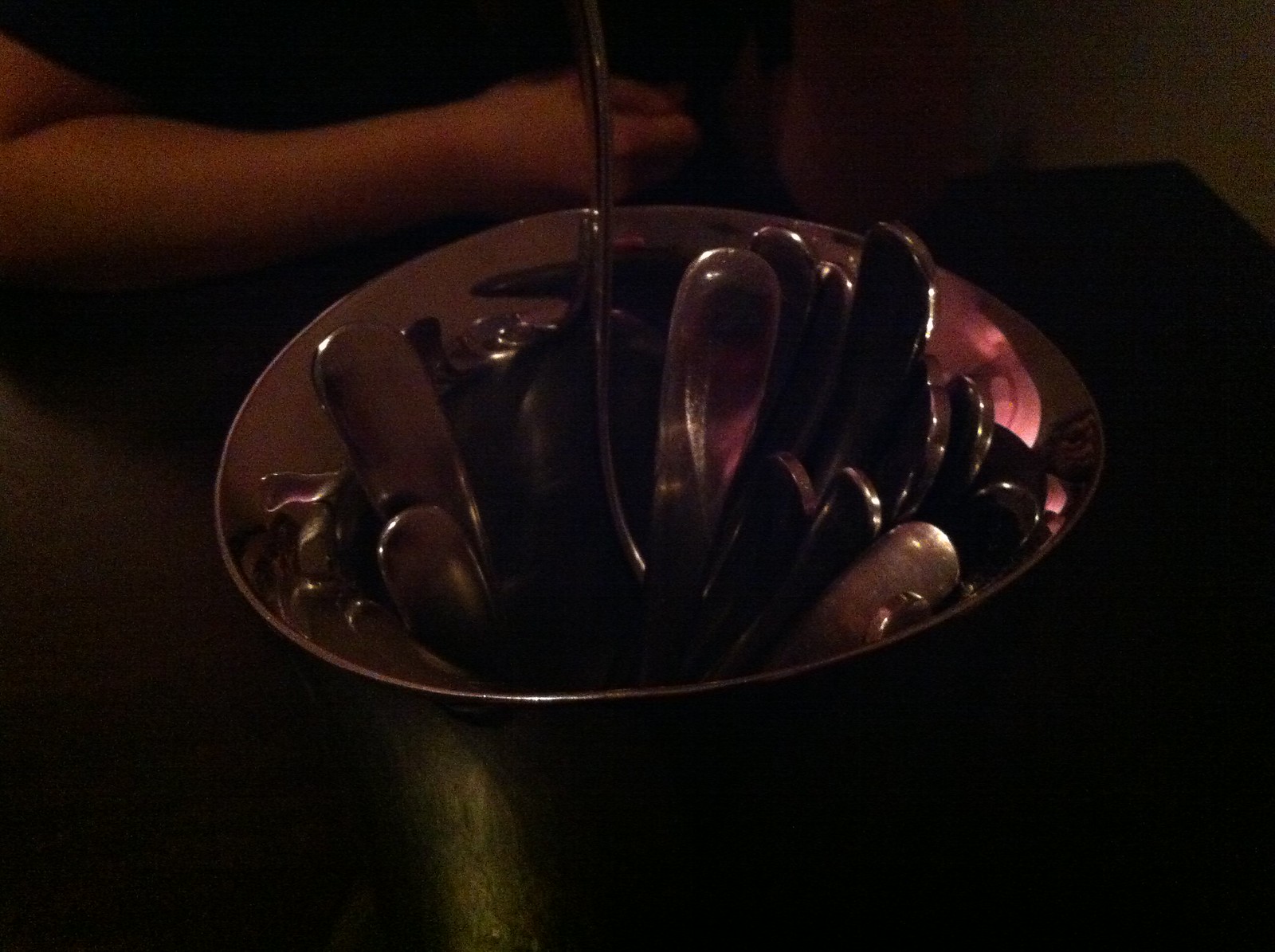In this photograph, an ambiguously defined, dimly lit setting—possibly a dimly lit home, bar, or restaurant—features a medium-sized, matte black metal bucket with a flared top. Positioned on a dark table, the bucket appears to hold a collection of polished, round metallic objects that resemble shoe horns or silverware, with some stones being brown or black. The bucket's center has an element that resembles a handle or a central fixture. The reflective surface of the bucket creates an optical illusion, initially making it look like a silver candy dish. In the background, we can discern the right arm of a person with beige skin, resting across their body, dressed in a dark shirt. The overall image is very dark, potentially highlighted by some subtle, pinkish mood lighting reflecting off the bucket. The rest of the surroundings fade into a near-uniform blackness, making it difficult to discern additional details.